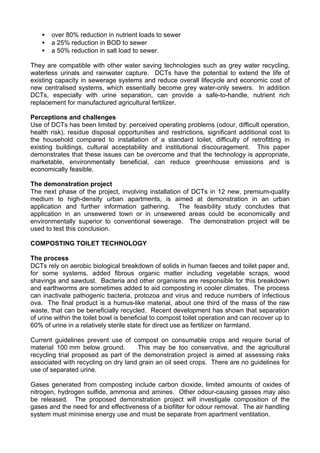The image features a detailed black-and-white text excerpt, seemingly taken from a textbook or manual, concentrating on composting toilet technology. It begins with a set of bullet points discussing significant reductions in nutrient loads, such as an 80% reduction in nutrient loads to the sewer, a 25% reduction in Biochemical Oxygen Demand (BOD), and a 50% reduction in salt load. The text highlights compatibility with other water-saving technologies like gray water recycling, waterless urinals, and rainwater capture.

Following the bulleted points, the text delves into various aspects of composting toilet technology. The "Perceptions and Challenges" section discusses the marketability, environmental benefits, greenhouse gas reduction, and economic feasibility of the technology. Another key section, "The Demonstration Project," outlines plans to install composting dry toilets (DCTs) in 12 new premium urban apartments. The core of the excerpt explains how DCTs rely on aerobic biological breakdown to decompose human feces, toilet paper, and produce gases like carbon dioxide, limited oxides of nitrogen, hydrogen sulfide, and ammonia.

Throughout the image, headings and subheadings structure the content, including a prominent header for "Composting Toilet Technology" and sections labeled "The Process." This structured format emphasizes the efficiency and multifaceted benefits of composting toilet technology, while also noting current guidelines that limit compost use.